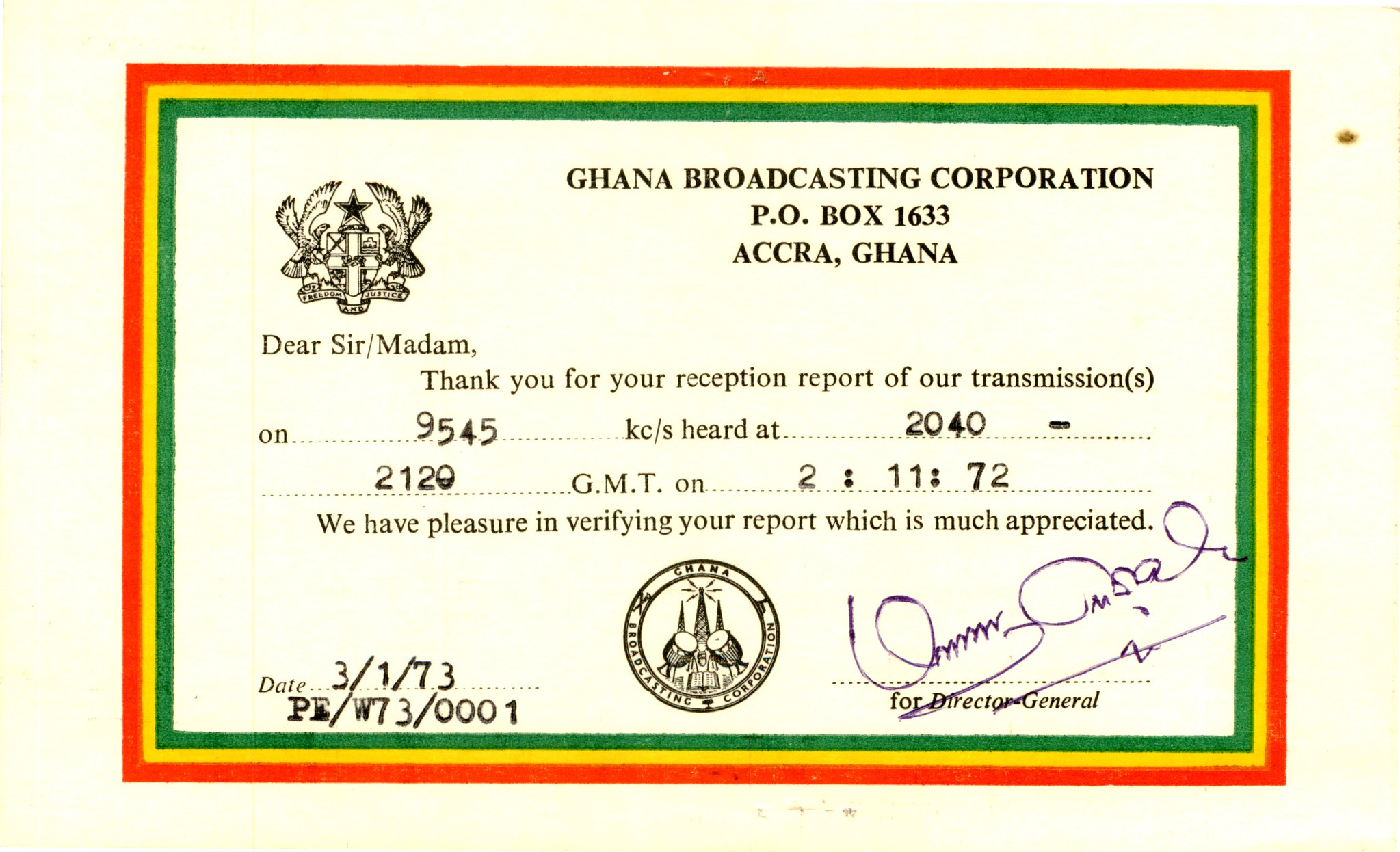The image depicts a rectangular verification card from the Ghana Broadcasting Corporation, bordered with three consecutive colors: red on the outermost edge, followed by yellow, and green on the innermost edge. At the top center of the card, it reads "Ghana Broadcasting Corporation, P.O. Box 1633, Accra, Ghana." In the upper left corner, there is a national emblem featuring a black star flanked by what appear to be eagles, symbolizing the country of Ghana. 

The main body of the card contains a formal message: "Dear Sir/Madam, thank you for your reception report of our transmissions on 9545 KC/S heard at 2040-2120 GMT on 2-11-72. We have pleasure in verifying your report, which is much appreciated." The date, 3-1-73, is noted on the lower left corner, followed by a reference code "P.E./W-73/0001." In the bottom right corner, the card is signed by the Director General, although the signature is indecipherable. 

At the center of the card, there is a circular emblem containing the text "Ghana Broadcasting Corporation" encircling the corporation’s symbol.